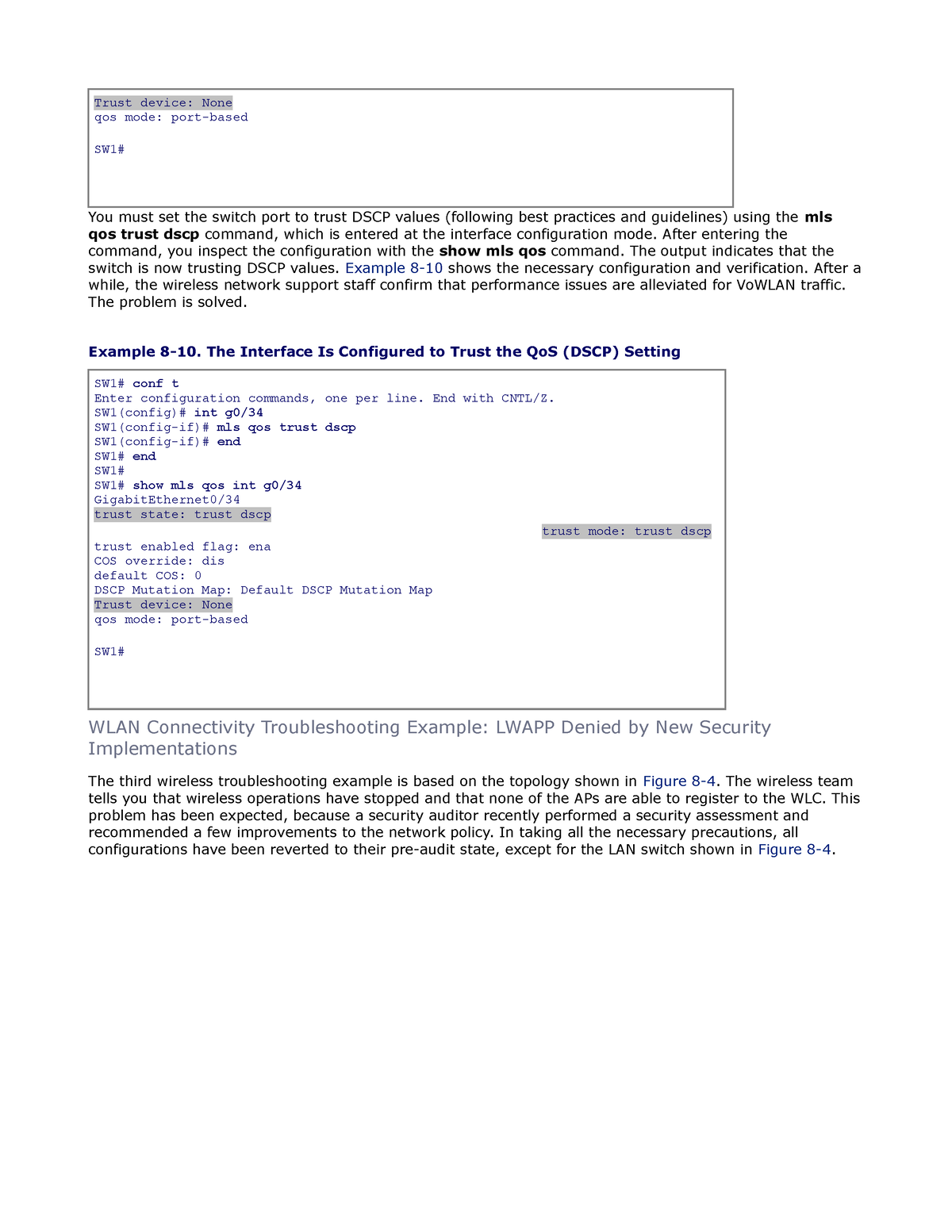- **Screenshot of a Networking Configuration Web Page**

The image is a screenshot of a web page displaying two distinct sections containing detailed networking configuration information. 

- **Top Section: QoS Configuration**

At the very top of the page is a box with a gray-highlighted line stating "trust device none." Below this, there is a section labeled "QoS mode" with the value "port-based," and the final row in this box reads "SW1#" followed by a brief explanatory text. The first sentence of this text, in bold, reads: "MLS QoS trust DSCP". The complete sentence instructs, "You must set the switch port to trust DSCP values using the MLS QoS trust DSP command, which is entered at the interface configuration mode."

- **Second Section: Example Configuration Code**

The second box is titled "Example 8-10" in blue text. This section shows an interface configured to trust QoS DSCP settings. Inside this box is a substantial block of code, more than 10 lines long, with specific fragments highlighted in gray. Notably, the terms "trust state" and "trust DSCP" are highlighted in gray, indicating their importance. On the far right, "trust mode" is also highlighted in gray. Near the bottom of this box, it is again noted that the configuration specifies "trust device none."

- **Additional Information: WLAN Connectivity Troubleshooting**

Below the second box, there is a section titled "WLAN connectivity troubleshooting example. LWAPP denied by new security implementations," followed by a detailed explanation. Most of this explanatory text is in black, with specific drawings rendered in blue. The label "figure 8-4" appears twice within the paragraph, also highlighted in blue.

This comprehensive description provides a clear and detailed understanding of the web page's content and the configuration examples it illustrates.